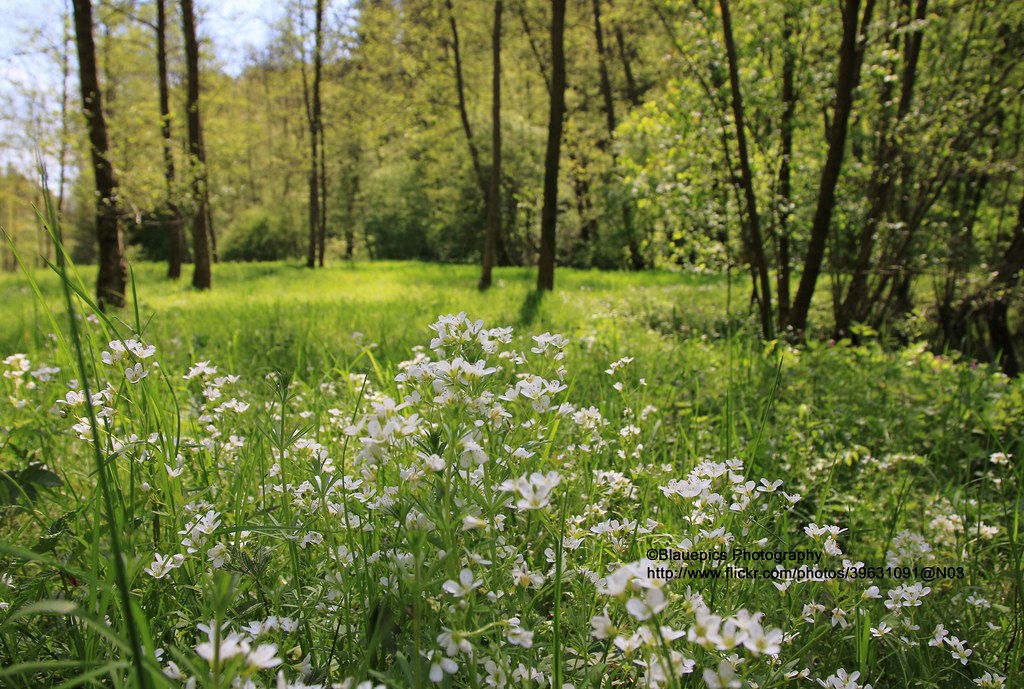The photograph, titled "Blaupix Photography," captures a vibrant daytime scene of a verdant meadow or forest edge, found on Flickr. Dominating the image, lush and vibrant green trees cast shadows across the landscape, interspersed with smaller growth trees that have long trunks and dense foliage. The forefront is adorned with tiny, delicate white flowers sprouting from tall grasses, their fine details in sharp focus. In contrast, the background offers a gentle blur of trees and grasses, adding depth to the composition. A sliver of light blue sky peeks through the upper left corner, enhancing the sense of a bright, sunny spring day. The bottom right corner of the image quietly features black lettering that reads "Blaupix Photography," followed by a URL: "http://www.flickr.com/photos/39631091@N08."